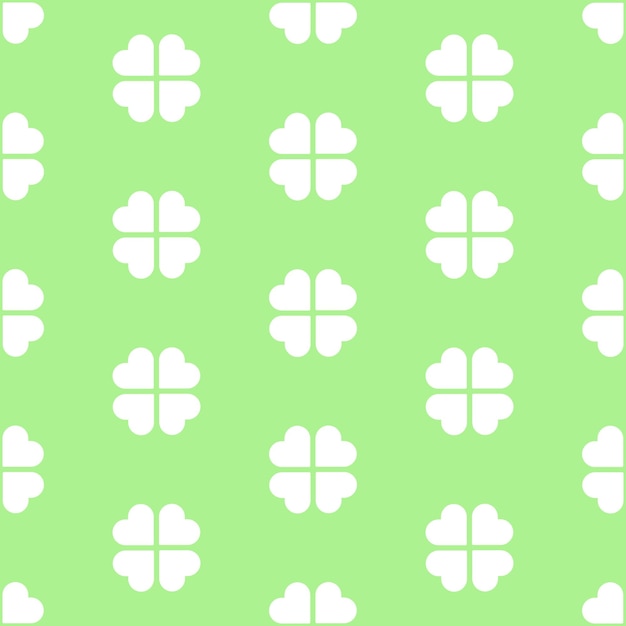The image is a square graphic featuring a repeating pattern on a light mint-green background with a thin, green border. The pattern consists of clover-like shapes formed by four hearts pointing inwardly toward each other, creating a green cross shape at the center of each clover. In the design, these clovers are arranged so that complete shapes appear in the corners and along the sides, while near the edges, only partial clovers can be seen, contributing fragmentary segments like single heart leaves. There are two full rows of complete clovers on the left and right sides, totaling four clovers per row, each evenly spaced. At the top center and bottom center of the graphic, there are two visible heart leaves, and in the middle of the design, three full clovers are arranged. The pattern is symmetrical and designed to tile seamlessly if duplicated.